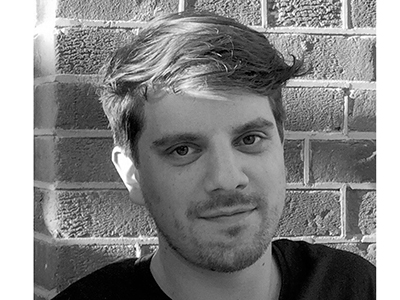The black and white photograph depicts a young Caucasian male, appearing to be in his early twenties. He has longish hair on the top that is shaved shorter on the sides, and it is swept over to the right side of the image. His facial features include dark eyes, dark eyebrows, and a stubble around his mouth and chin, with a slight moustache indicative of a recently shaved beard. He is dressed in a dark-colored top, likely a black sweater or t-shirt with a ring neck. The background features a brick wall with light-colored grout, adding texture to the scene. The lighting in the image suggests sunlight coming from the left, casting shadows and illuminating his hair, contributing to the overall textured and detailed composition. His expression is a subtle grin, looking directly at the camera, but framed in a three-quarter angle shot that reveals a bit of his right ear.